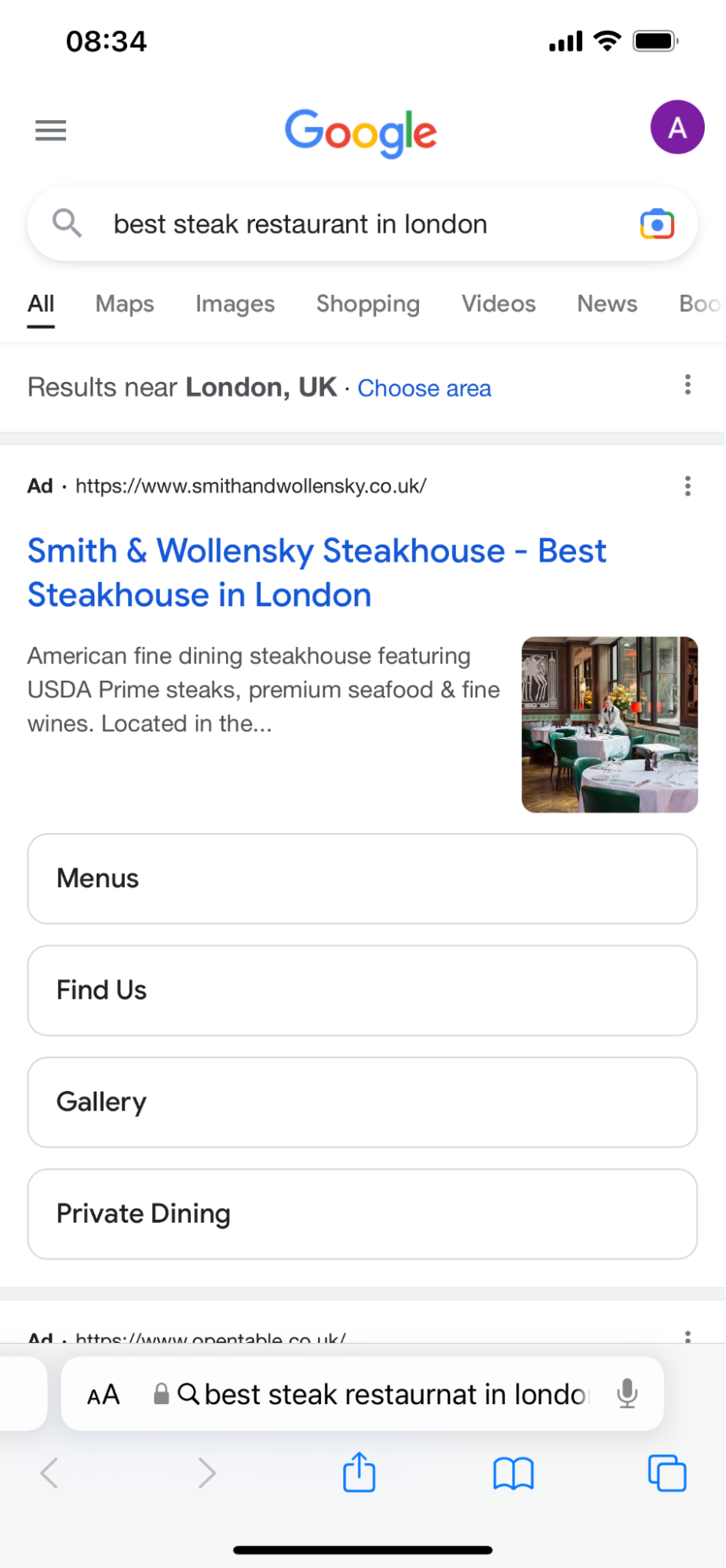The image displays a Google search results page. At the top left, the time is indicated as 8:34. Moving to the right are icons for connectivity, Wi-Fi, and battery percentage. Below, the Google logo is prominently featured with a purple profile icon containing an "A" to the right and a tab menu icon to the left.

Centered beneath these is a search bar, with the query "Best Steak Restaurant in London." Directly below the search bar, categories are listed: "All" (highlighted), "Maps," "Images," "Shopping," "Videos," and "News," with the last category being obscured. The section underneath reads "Results near London, UK," followed by a blue link that says "Choose Area."

The first search result, marked with an "Ad" label, is a link to the Smith & Wolensky Steakhouse, featuring the text "Best Steakhouse in London" in blue. There is an accompanying image of the restaurant's interior in the bottom right corner of the ad. Categorized links in black text follow: "Menus," "Find Us," "Gallery," and "Private Dining."

Finally, the search bar at the bottom of the screen again shows "Best Steak Restaurant in LONDO" in incomplete form. Below this bar, five icons are displayed: left and right arrows, a share icon in the center, a bookmark icon, and a tabs icon on the far right.